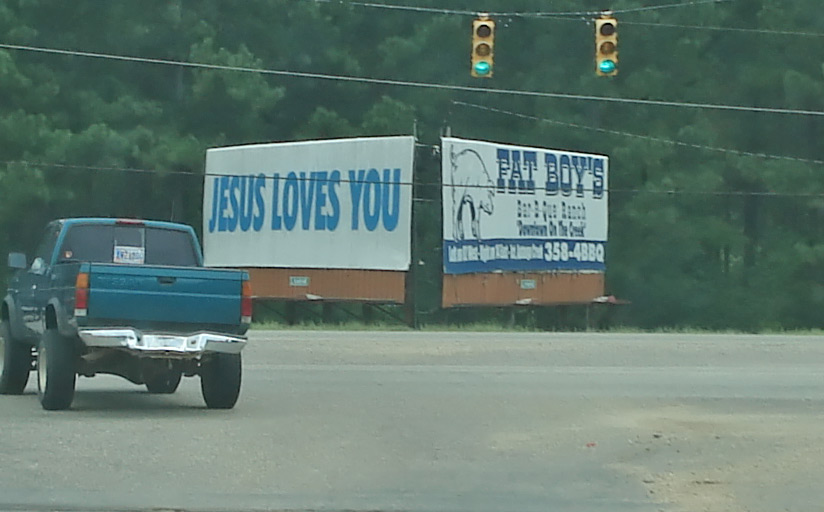In this image, there is a high road intersection featuring two illuminated green stoplights hanging above. To the left of the intersection, a greenish-blue pickup truck is visible, showcasing red and orange taillights and a bright silver bumper, with tires that extend slightly beyond the fenders. Positioned in the background is a tree line of deep green trees, enhancing the natural setting. Dominating the center of the image are two white billboards forming a V shape. The left billboard, with blue print, reads "Jesus Loves You" and features a grayish-orange band at the bottom. The right billboard also displays blue print, advertising "Fat Boys Barbecue Ranch, Downtown on the Creek, 3584 BBQ" along with a silhouette of a pig. The convergence of natural and urban elements creates a contrasting yet harmonious scene.